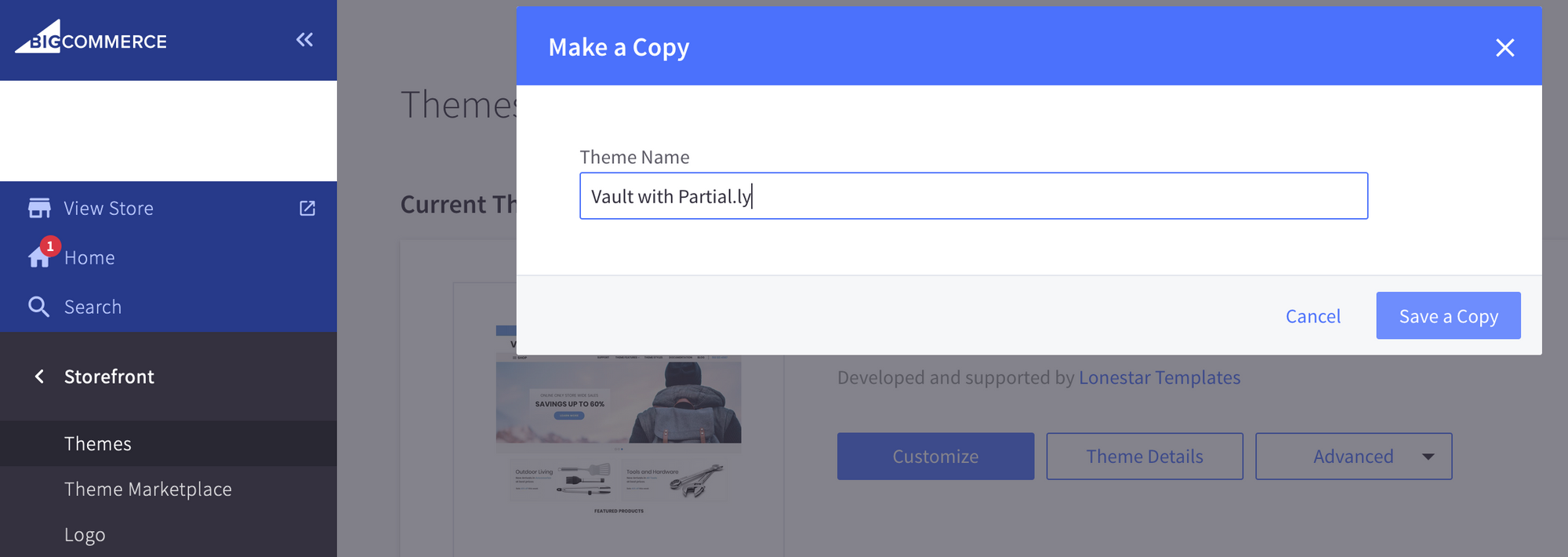This image is a detailed screenshot with a horizontal rectangular layout, prominently featuring the BigCommerce interface. In the top-left corner, there is a blue box with the words "BigCommerce"; "Big" is rendered in blue text within a white triangle, while "Commerce" is in white text. Directly below this, there's a narrow white banner.

Underneath, there's another blue box containing navigation options: "View Store," "Home" (which has one unread message notification), "Search," and below these, a black box with "Storefront" written in white text. Further down, the interface lists options such as "Themes," "Theme Marketplace," and "Logo."

To the right of these options, there's an open white box occupying a significant portion of the image. This box is topped with a blue banner or header that reads "Make a Copy" in white text, accompanied by a white "X" on the right side for closing the banner. Below this header, the box has a white background, with a prominent blue box that says "Vault with Partial.ly" in black text. Above this section, "Theme Name" is indicated.

The image captures various elements and navigation tools within the BigCommerce platform, showcasing a detailed interface layout designed for managing online store themes and settings.